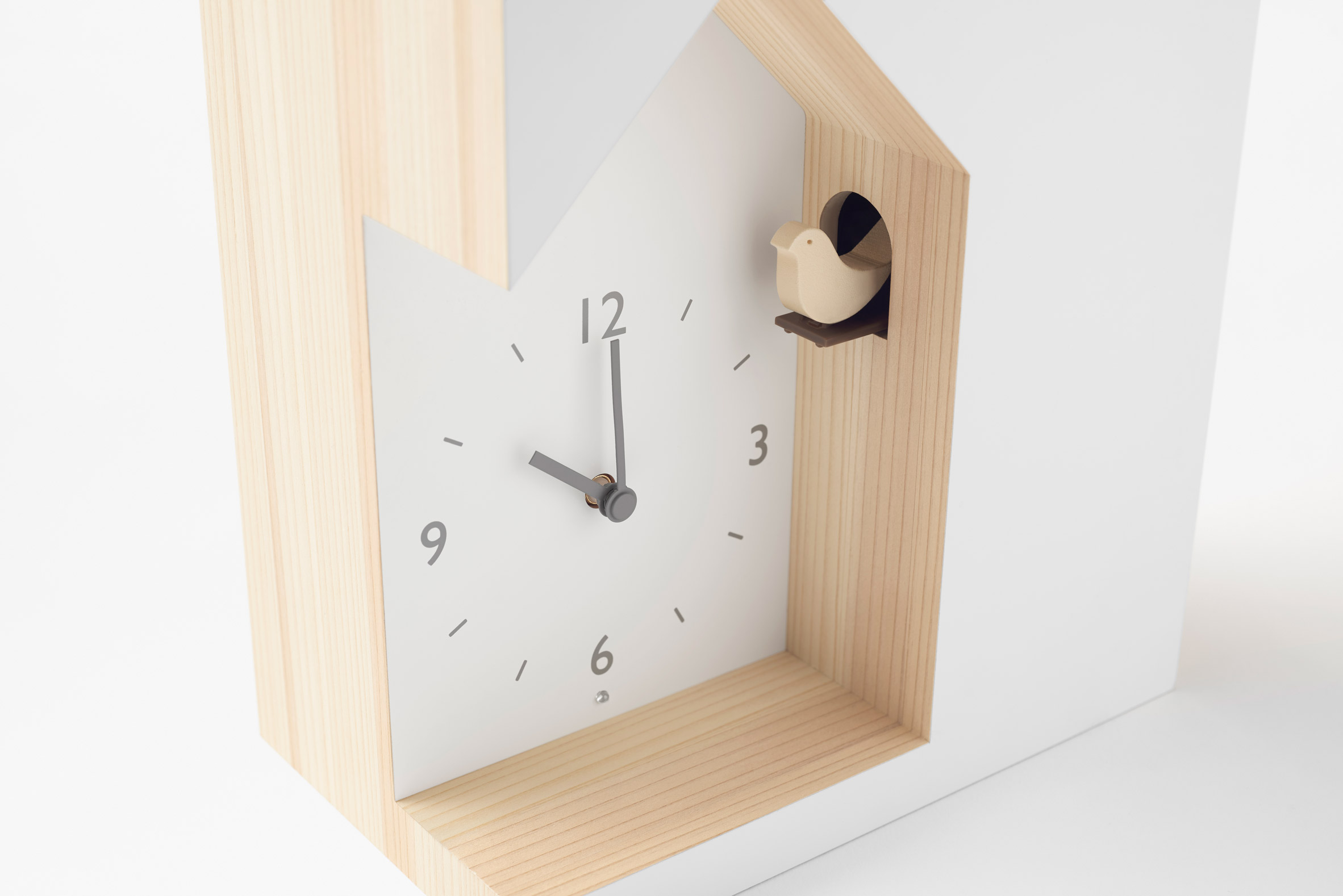The photograph features a minimalist, modern cuckoo clock set against an all-white background. This clock is characterized by its clean lines and the combination of white and pine-colored wood. Rectangular in shape with a distinctive house-like carving, the clock face is gray and only displays the numeral hours at 12, 3, 6, and 9. The remaining hours are represented by simple lines. The clock's silver-gray hour and minute hands stand out against the face. On the right side, there is a small arch-like opening made from the same wood material, where a bird toy perches, adding a charming, integrated element. The overall design is reminiscent of a product you might find at IKEA, with its simplicity and contemporary aesthetic. The time displayed on the clock is precisely 10 o'clock.